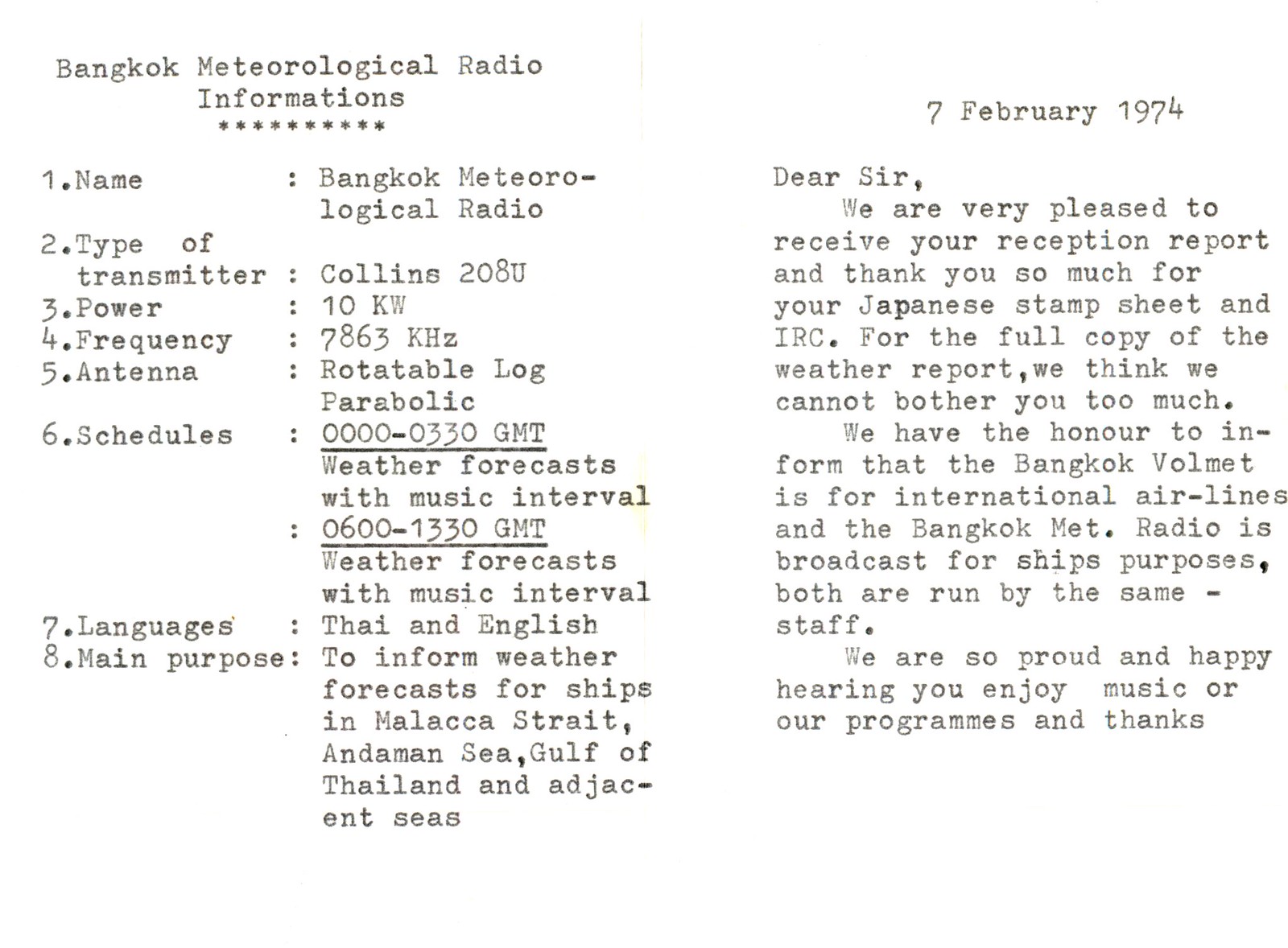The image features a typewritten report on a white piece of paper, dated 7 February 1974, titled "Bangkok Meteorological Radio Informations." The document is split into two sections. On the left, it details technical specifications and broadcasting schedules for the Bangkok Meteorological Radio. It lists:

1. **Name:** Bangkok Meteorological Radio
2. **Type of Transmitter:** Collins 208U
3. **Power:** 10 kW
4. **Frequency:** 7863 kHz
5. **Antenna:** Rotatable log-parabolic
6. **Schedules:**
    - 0000-0330 GMT: Weather forecast with music intervals
    - 0600-1330 GMT: Weather forecast with music intervals
7. **Languages:** Thai and English
8. **Main Purpose:** To inform weather forecasts for ships in the Malacca Strait, Andaman Sea, Gulf of Thailand, and adjacent seas.

On the right side, there is a letter addressed to a recipient, expressing gratitude for a reception report and the Japanese stamp sheet and IRC. The letter explains that the complete weather report cannot be provided, clarifies the distinction between Bangkok Volmet (for international airlines) and Bangkok Met Radio (for ship purposes), both managed by the same staff, and conveys happiness that the recipient enjoys the music programs.